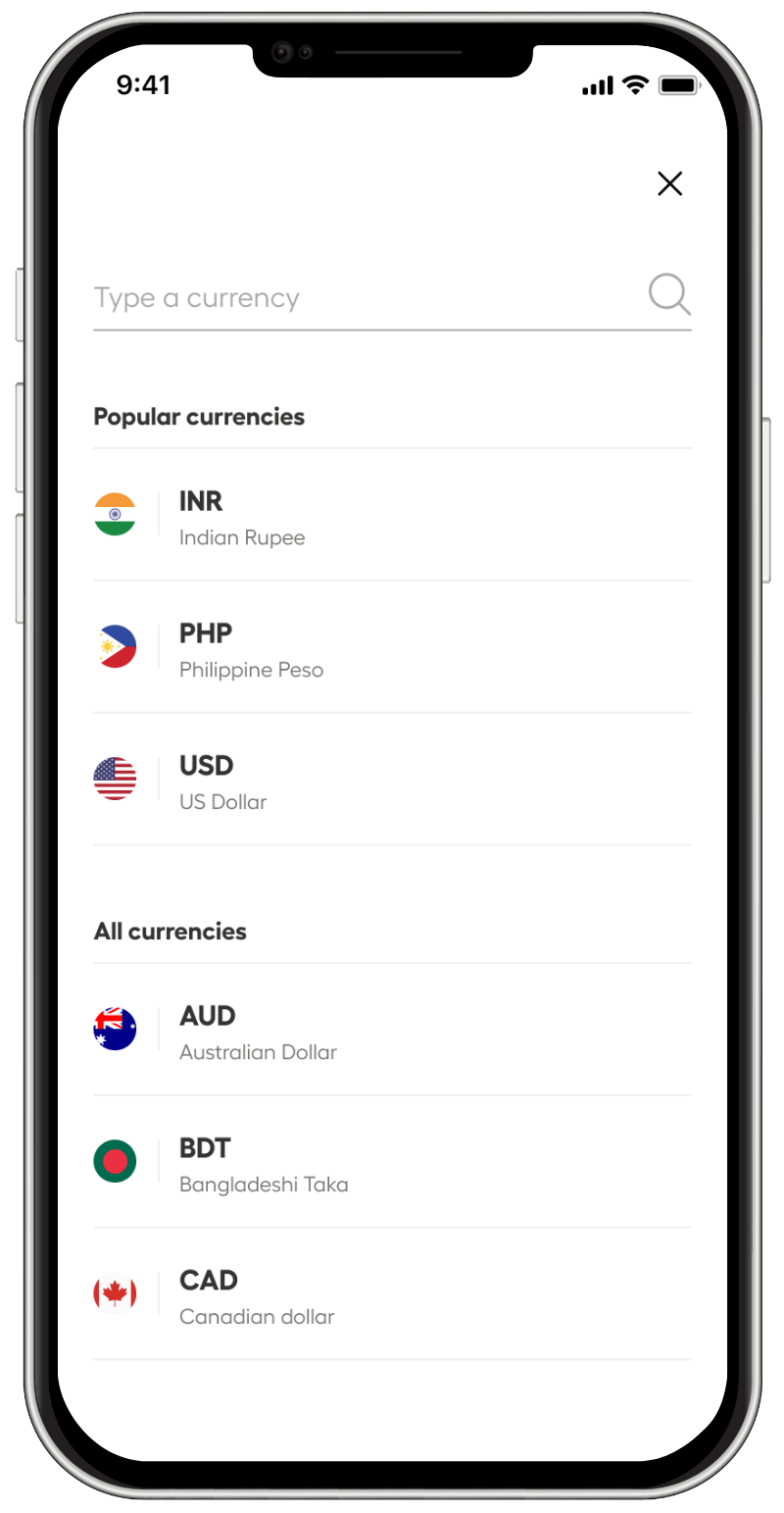In this image, we observe a detailed screenshot of a smartphone display featuring a currency search interface. At the top right corner of the screen, the battery icon is fully charged, indicating a full battery. Adjacent to this, the phone signal strength icon shows full bars, and the WiFi signal strength icon is also fully filled. The current time displayed on the top left corner is 9:41.

In the center at the top, there is a gray-colored search bar with the text "Type a currency" inside it. On the far right end of this search bar is a magnifying glass icon, also in gray. Just below the search bar, the heading "Popular Currencies" is prominently displayed in black text.

Under this heading, three currencies are listed: the Indian Rupee, Philippine Peso, and US Dollar. Each of these listings is accompanied by their respective national flags. The Indian flag features stripes of orange, white, and green. The Filipino flag contains colors white, blue, and red. The American flag displays its iconic colors of blue, white, and red.

Following this section, the text "All Currencies" appears, suggesting a comprehensive alphabetical list of currencies below. Only three currencies are visible in this screenshot: Australian Dollar, Bangladeshi Taka, and Canadian Dollar.